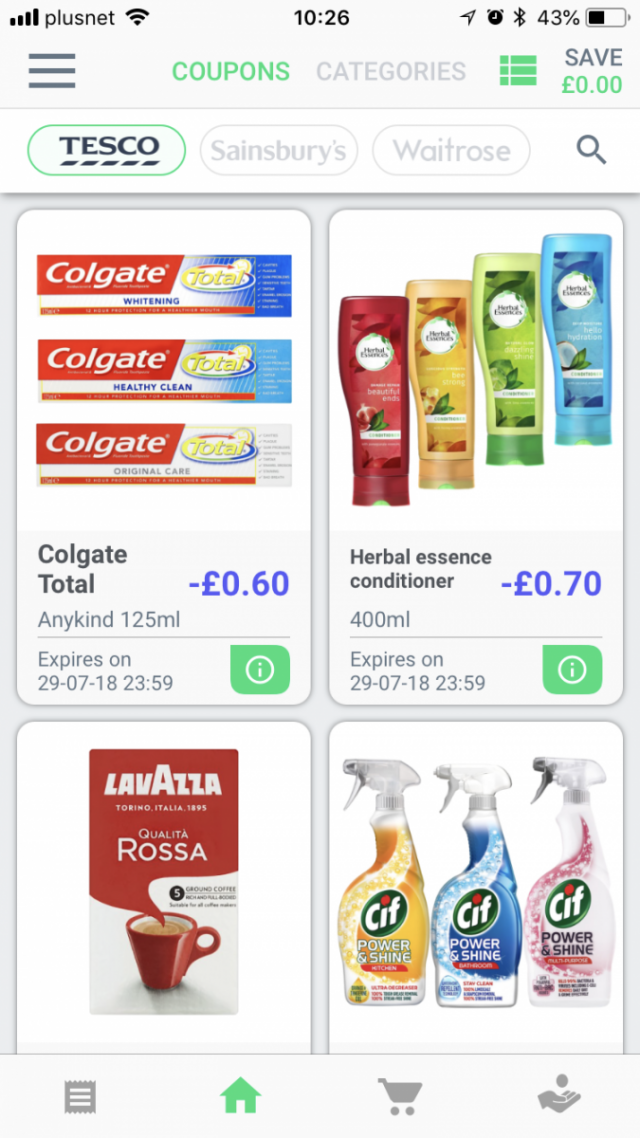Screenshot of a mobile phone screen displaying various app icons and status indicators at the top, including four bars of signal strength, Wi-Fi connection, time (10:26), 43% battery, active Bluetooth, and a Telegram notification. The app interface shows an e-coupons or deals section labeled "Coupons and Categories." 

Within this section, there are listings for different products. The first listing is for Colgate Total toothpaste, showing an image with three packs of 125ml toothpaste tubes. The deal offers a discount of 60 pence, expiring on 29/07/18 at 23:59. Below this offer is a green button with a lowercase 'i' inside a circle, presumably for more information.

Beside this, there is another section showing four plastic bottles of Herbal Essences conditioner in red, orange, green, and blue variations. This deal offers a discount of 70 pence on 400ml bottles, also expiring on 29/07/18 at 23:59, accompanied by another green information button.